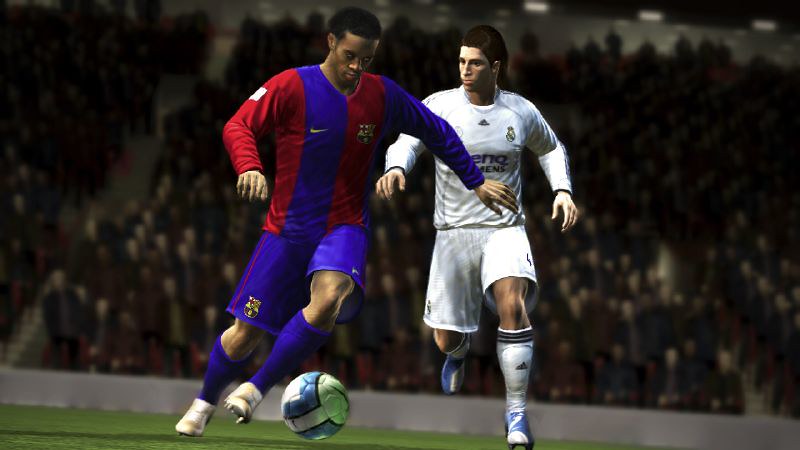The image is a detailed still from a soccer video game capturing an intense moment between two players vying for control of a soccer ball. The player on the left is slightly ahead and appears to be about to kick the ball. He is dark-skinned and wearing a blue and red vertically striped long-sleeve jersey with knee-length royal blue shorts. His attire also includes blue socks and white shoes. His right arm is extended straight back as if to stabilize or perhaps push the other player, while his left knee is bent upwards in motion. The player on the right, who has light skin and dark hair, is dressed in an all-white uniform featuring a black logo in the center of the shirt and black striped socks paired with blue and white shoes. He is running forward with both arms slightly out at his sides. The soccer ball they are contesting is primarily blue and green with a distinct white stripe and a green Nike swoosh. In the background, the crowded bleachers are blurred but clearly filled, creating a vibrant atmosphere. The image also shows a concrete barrier or divider along the stands and a patch of grass in the bottom left corner.